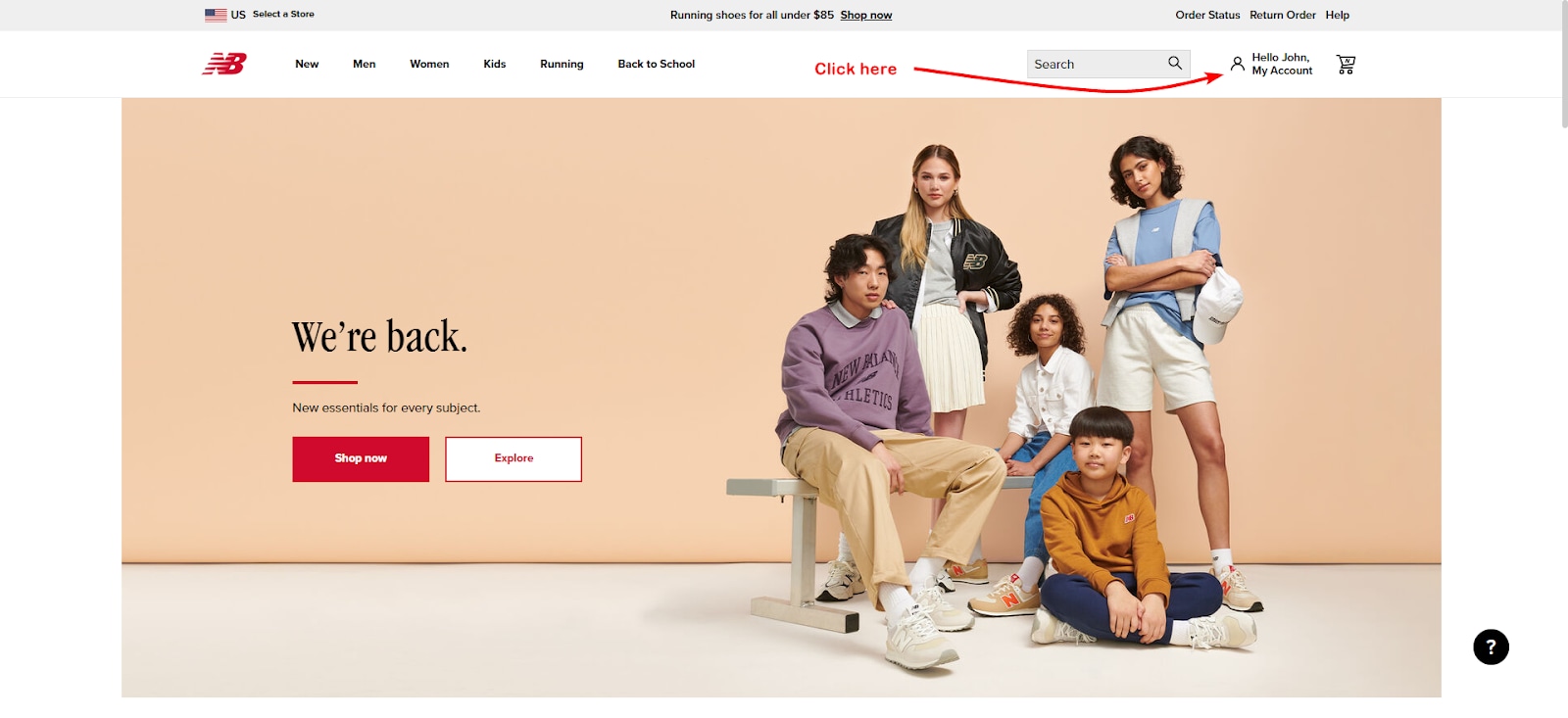The screenshot captures a detailed view of a website's homepage, featuring a structured and user-friendly layout. The topmost section is a light gray header that spans the width of the page. Positioned on the left side of this header is an American flag icon, directly adjacent to uppercase black text reading "US." Moving rightwards—and slightly upward—is dark gray text that prompts the user to "Select a Store."

Centered in the header, amidst ample negative space, appears bold dark gray text stating, "Running shoes for all under $85" followed by an underlined "Shop now" call to action. In the top right corner, you’ll find another set of gray text, listing "Order status," "Return order," and "Help," each separated by subtle spacing.

Below this header, a white secondary header displays prominently. On its left side rests the brand’s logo, a stylized red "NB" comprised of horizontal red lines forming the letter "N." Immediately to the right of the logo, a navigation menu in gray text lists categories sequentially: "New," "Men," "Women," "Kids," "Running," and "Back to School."

Particularly striking is the overlay in red text, situated between "Back to School" and the search bar. It commands attention with the phrase "Click Here," directing users visually with a smooth, long red arrow pointing towards the profile picture icon located just right of the search bar.

A light gray search bar, placed to the right of the navigation menu, features placeholder text "Search" on its left and a dark gray magnifying glass icon on its right. Adjacent to this, a gray profile picture icon sits atop two lines of dark gray text that greet the user: "Hello, John" and "My Account." Farther right is a dark gray shopping cart icon.

Beneath these headers lies the main body of the homepage. It features an engaging image of five individuals alongside a few interactive buttons, completing the informative yet visually pleasing layout of the homepage.